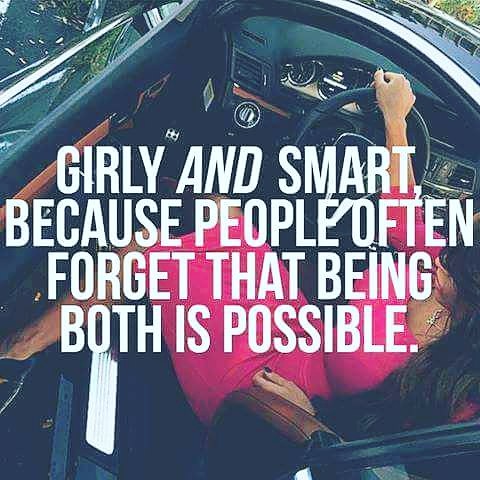In this vibrant internet meme, a young woman with long dark hair sits confidently in the driver's seat of a designer luxury car, her pink knee-length dress and matching high heels adding a touch of elegance. The photograph, captured in color from an elevated perspective, shows her right hand on the steering wheel and her left leg extended out of the open car door, hinting at both arrival and departure. The background reveals hints of grass, emphasizing the outdoor setting in broad daylight. Dominating the image is the prominent superimposed text, "Girly and smart because people often forget that being both is possible," underscoring the meme's empowering message. The car's interior details, including the control panels, are visible, though the make and model remain indistinct.